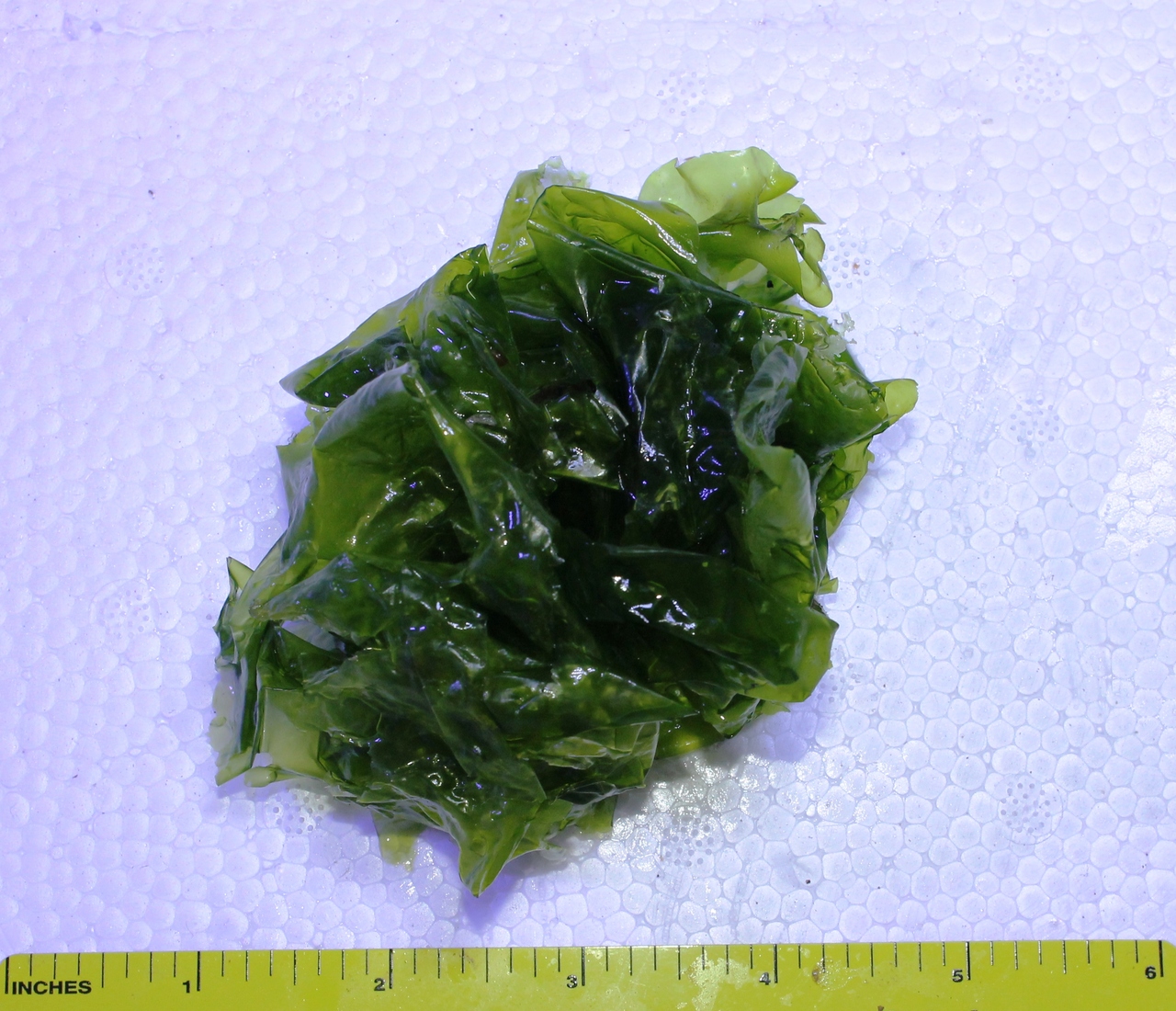The image showcases a dark green, crumpled object that strongly resembles seaweed or possibly steamed spinach, lying on a white, dotted surface which might be covered in small white crystals. The object, appearing shiny and wet with lighter green edges and a dark green, almost black center, is about 4 to 4.5 inches long and around 2 inches wide. Below this mysterious vegetable-like item, a measuring tape is laid out horizontally in inches, extending from 0 to 6 inches. The green object spans from the 1-inch to the 4.5-inch mark and is positioned just above, not directly on, the tape measure. The precise lines and markers on the measuring tape emphasize the scale of the object, highlighting its detailed dimensions.